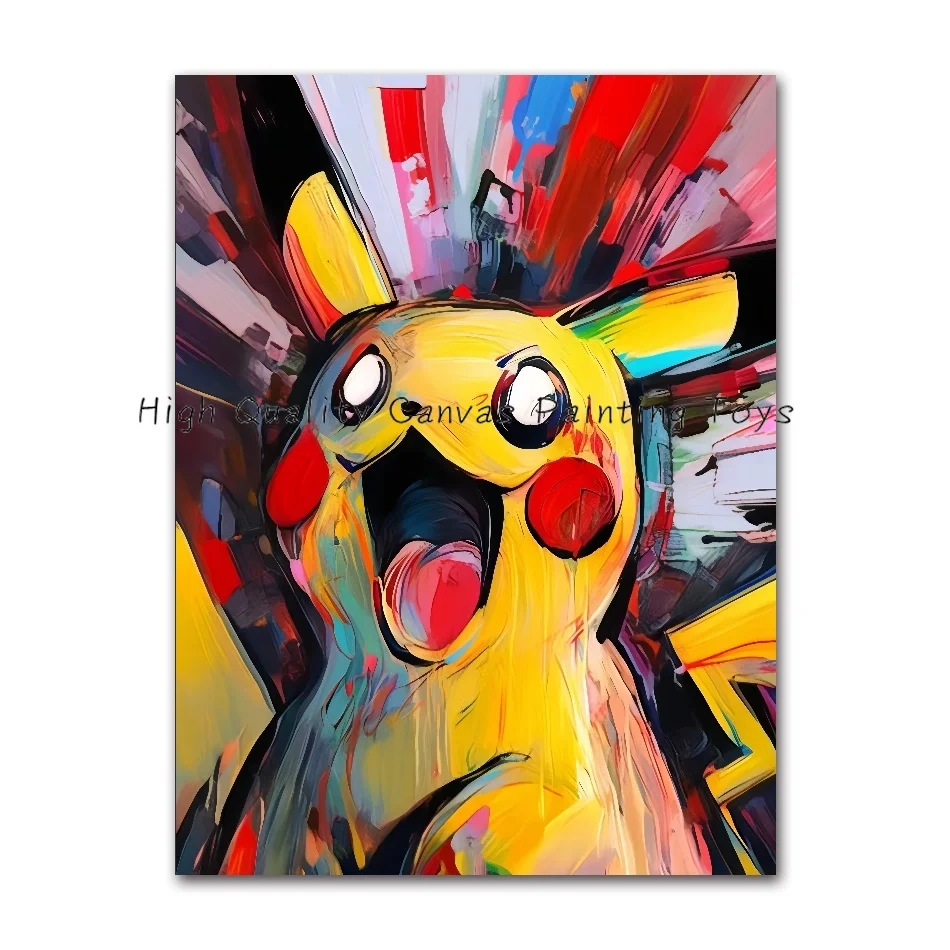This vivid watercolor painting features Pikachu, the iconic Pokémon, but with a surreal twist. Pikachu is prominently placed in the center, its normally cheerful features now more intense and abstract. Its mouth is wide open in what appears to be a yell or an excited expression, with its tongue visible inside. Pikachu's typically vibrant yellow fur is accentuated with unexpected hues of blue, green, and pink. The familiar red circles on its cheeks stand out against its face, but its eyes are unsettlingly white, adding to the surreal atmosphere of the piece.

The background is equally dynamic and chaotic, featuring swirling, bold light flares and stripes in a mix of reds, blues, blacks, grays, and whites, creating a sense of rapid movement. This chaotic blend of colors seems to envelope Pikachu, contributing to the overall energetic and somewhat frantic feel of the painting. Pikachu's tail can be seen angled and prominent amidst the chaos, reinforcing its recognizable form despite the abstract stylings. The watercolor technique blurs and melds the colors, making the entire composition both captivating and slightly disorienting.